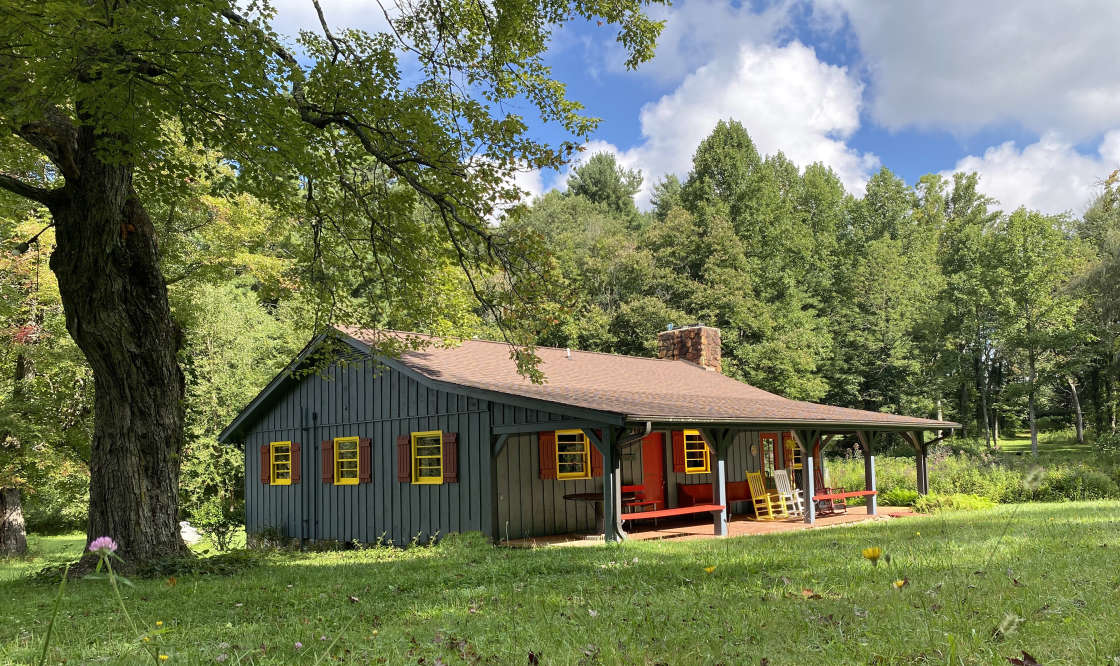The image features a quaint single-story cabin nestled in a lush, verdant landscape, likely part of a farm or woodland setting. The cabin, rectangular in shape, is clad in vertical dark gray wood siding with red shingles on its roof and a prominent red-brick chimney protruding from the right side. The house's windows are adorned with yellow frames and red storm shutters, and it boasts a bright red front door. Clusters of fallen leaves and a sprinkling of dandelions are noticeable on the expansive green lawn that extends in front of the cabin. A charming porch runs the length of the house, supported by five pillars, offering shelter under an overhang. Situated on this porch are two inviting rocking chairs, one painted white and the other yellow. Adjacent to the cabin on the left stands a large, old tree with a curving trunk and abundant green leaves. Beyond the house, a dense ring of trees with lush foliage forms the backdrop, under a sky with a mix of blue and gray clouds.